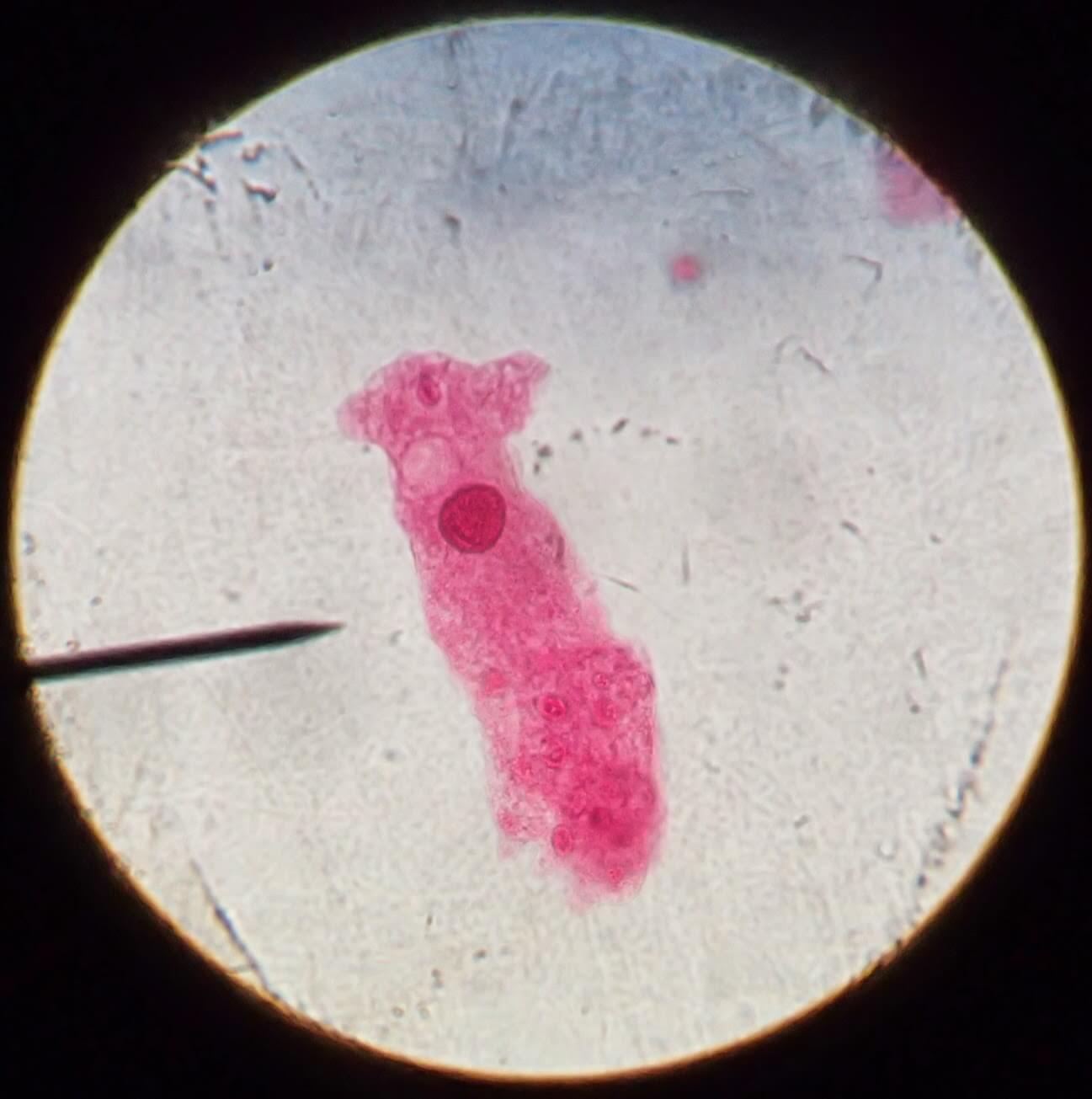This detailed image, captured through a microscope, showcases a cellular structure at high magnification. The photograph is framed by a black circular border, a common feature of microscopic imaging. At the center, a pink-hued cell, with a deeper red nucleus, stands out prominently. The cell itself is somewhat oval with a protrusion on the upper right, resembling a beak, giving it a bird-like appearance. The background of the image is speckled with rough marks and scuffs, possibly indicating the texture of the slide or surrounding medium. A fine pin, visible entering from the left middle side, appears poised to interact with the cell, either for prodding or dispersing purposes, highlighting the specimen's meticulous examination in the lab.